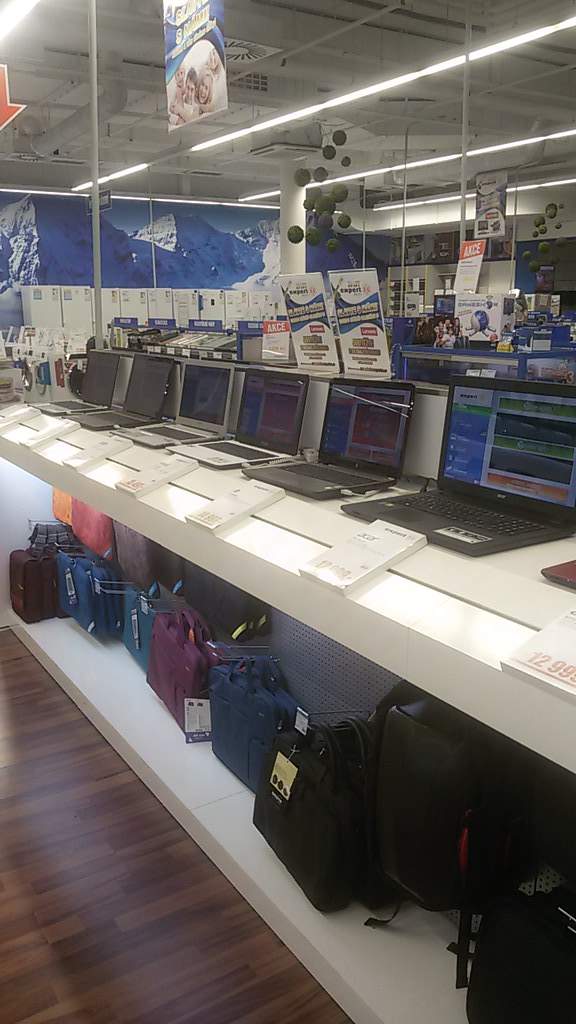The image is taken inside an electronics store, possibly a smaller outlet like a Best Buy but named "A-K-C-E," which suggests it might be a European or foreign store. In the foreground, there is a bright white counter with six open laptops lined up in a row. Each laptop features a Foamcore sign displaying prices, including figures like 12,995 or 12,999. The laptops come in various colors, with black, gray, silver, and white models visible.

Beneath the countertop, there is an open shelf that holds an array of laptop bags and carriers in different colors like black, blue, turquoise, purple, brown, and orange. These are neatly arranged on a pegboard wall, hanging from small arms extending out.

The store has a brown wood grain floor and the room is well-lit with fluorescent lights. On the back wall, there's a large mural depicting snow-covered mountains, which adds a scenic touch to the high-tech setting. Above, the open ceiling reveals ductwork, air conditioning vents, and rows of light fixtures. Additionally, there are circular mobiles or round decorations hanging from the ceiling, in dark gray to green colors. The background includes white refrigerators and other electronics on display, emphasizing the store's diverse range of products.